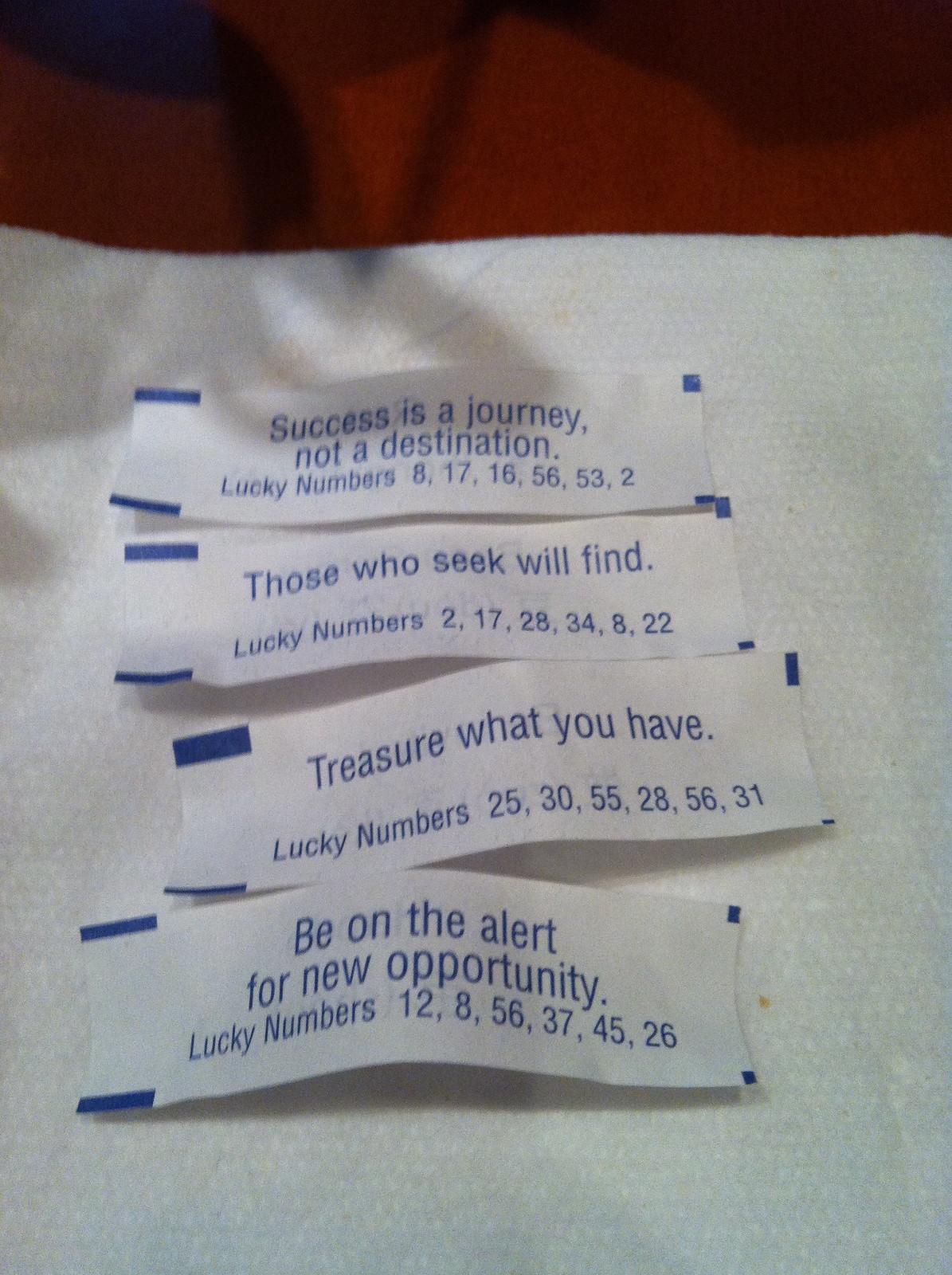This color photograph captures four fortune cookie fortunes arranged sequentially from top to bottom on a white napkin, which is placed on a red tablecloth. The fortunes are displayed in the following order: The top fortune reads, "Success is a journey, not a destination," followed by the lucky numbers 8, 17, 16, 56, 53, and 2. The second fortune states, "Those who seek will find," with the lucky numbers 2, 17, 28, 34, 8, and 22. The third fortune advises, "Treasure what you have," accompanied by the lucky numbers 25, 30, 55, 28, 56, and 31. The final fortune says, "Be on the alert for new opportunity," with the lucky numbers 12, 8, 56, 37, 45, and 26.